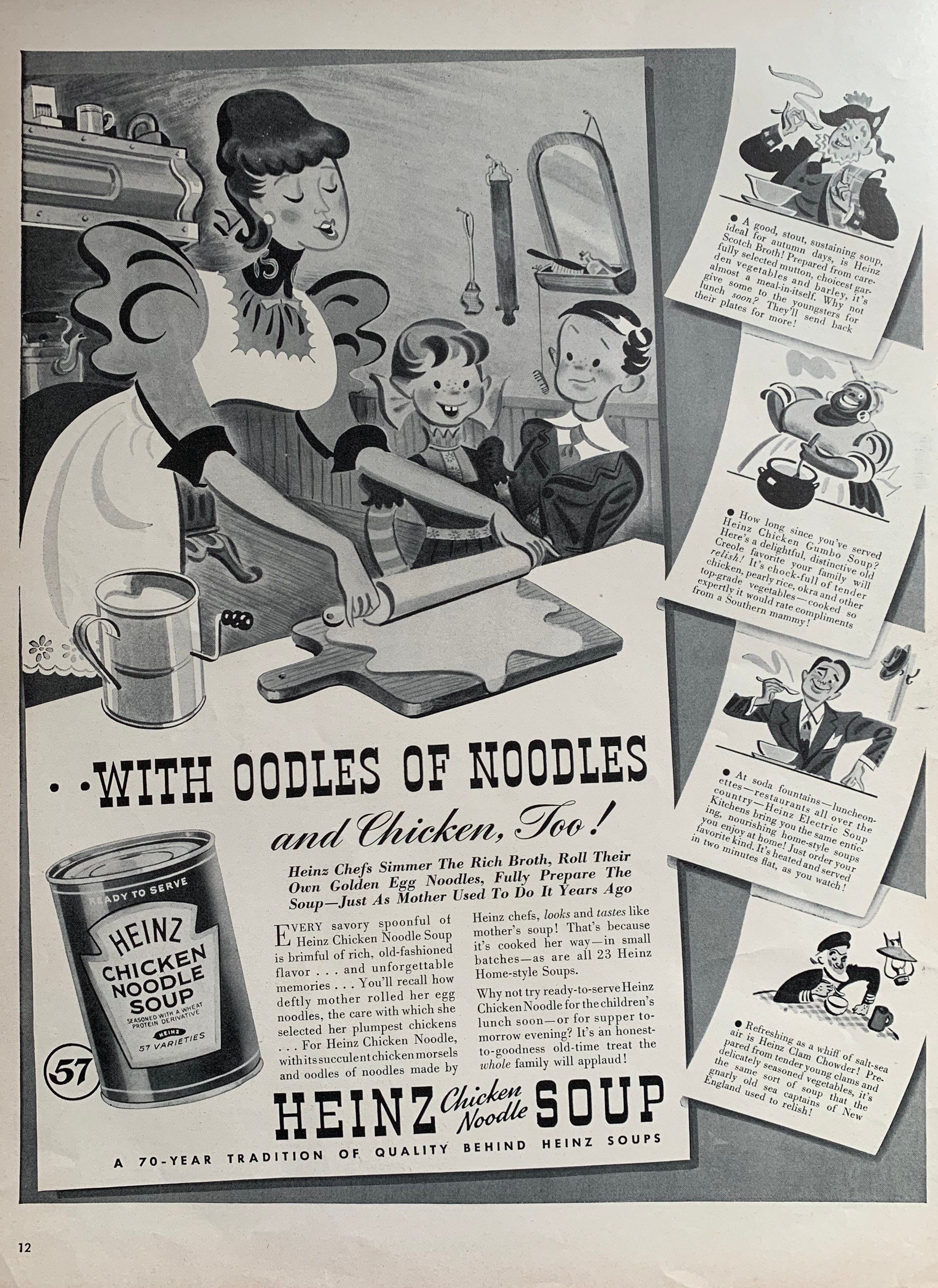This vintage magazine advertisement features a charming 1950s-style cartoon illustration of a woman in a frilled-shoulder dress and apron, happily rolling out dough with a rolling pin on a cutting board. Her brown hair is neatly styled, and her eyes are closed in a contented expression. Her two children, a little girl with boxy, striped sleeves and a black dress on the left, and a little boy in a suit with parted hair on the right, watch attentively. Surrounding them, the background includes a mirror and hanging trinkets that give a homely feel.

Prominently displayed in the advertisement is the text: "With oodles of noodles and chicken too," emphasizing the hearty ingredients of Pines Chicken Noodle Soup. The ad continues to explain, in somewhat aggressive text, the rigorous efforts of Pines’ chefs: "Heinz chefs simmer the rich broth, roll their own golden egg noodles, fully prepare the soup, just as a mother used to do it years ago. Every savory spoonful of Heinz Chicken Noodle Soup is a rimful of rich old-fashioned flavor and unforgettable memories." The ad highlights the 70-year-old tradition of quality behind Heinz Soups, emphasizing the product's heritage and the comforting memories it evokes.

At the bottom, it boldly reads, "Heinz Chicken Noodle Soup," accompanied by nostalgic black-and-white photographs that might depict different family members or iterations of the brand's legacy, tying everything back to a cherished and time-honored tradition.